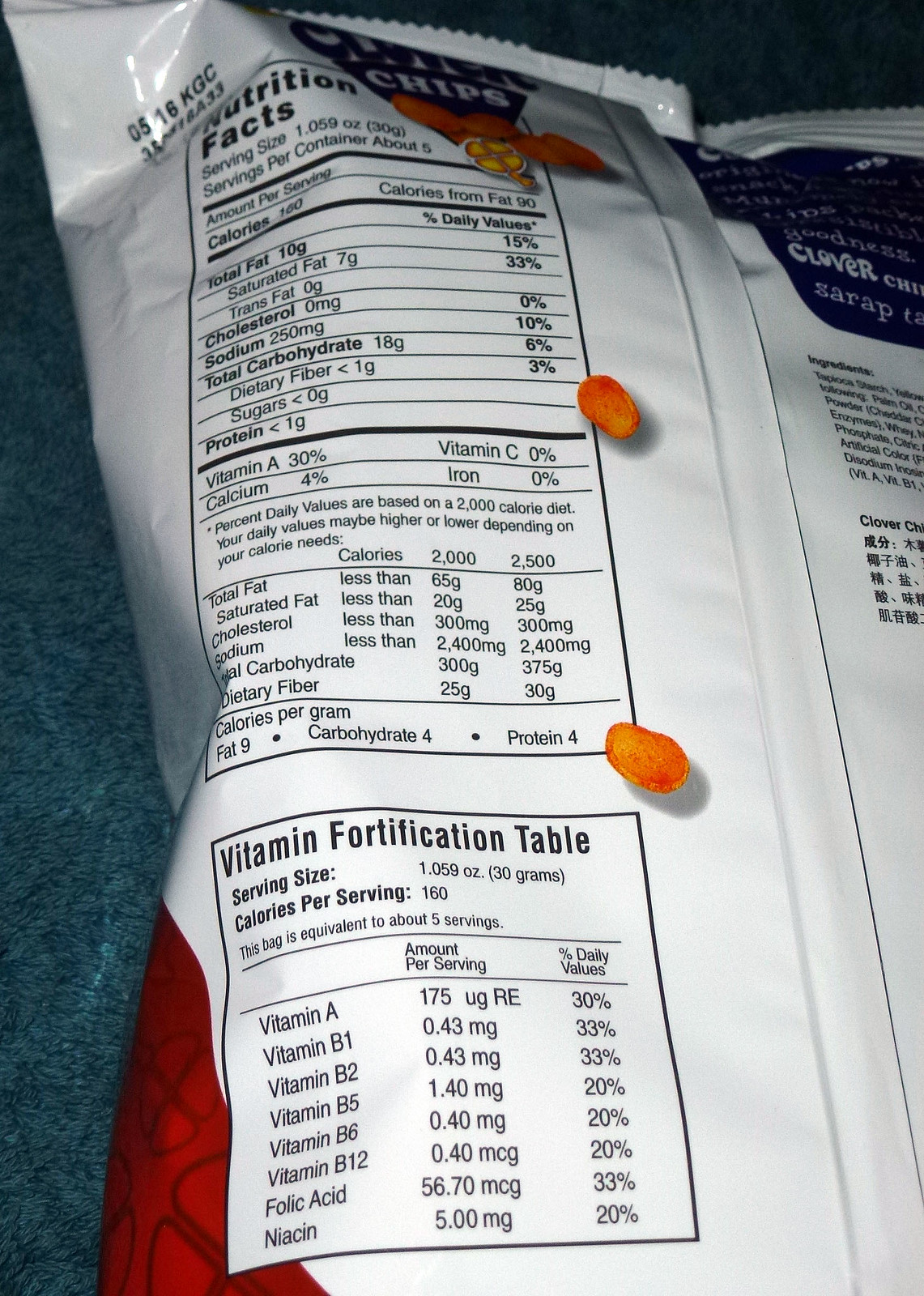This image showcases the back of a white plastic bag of chips with detailed nutritional information against a blue carpeted background. The top part of the bag features a date label "0516 KGC" and an obscure triangle-shaped logo. Below, in a blue section, the word "chips" is displayed prominently with no specific brand name, alongside two images of orange, puff-like chips, suggesting a possible cheese flavor.

On the left side of the bag, the nutrition facts are listed meticulously, stating the serving size of 1.059 ounces (30 grams) with about five servings per container. Detailed nutritional values are noted, including 180 calories per serving, 10 grams of total fat, and significant vitamin fortifications like 30% Vitamin A. Below the nutrition facts, a vitamin fortification table reiterates these values, specifying vitamins A, B1, B2, B5, B6, and B12, along with their respective daily values.

The lower left corner of the bag is marked with a touch of burgundy color. Additionally, a comprehensive ingredients list is located on the right side under another blue section. The composition of the image is focused on the informative aspect of the chips, highlighting the nutritional content and the visual appeal of the orange chip images.